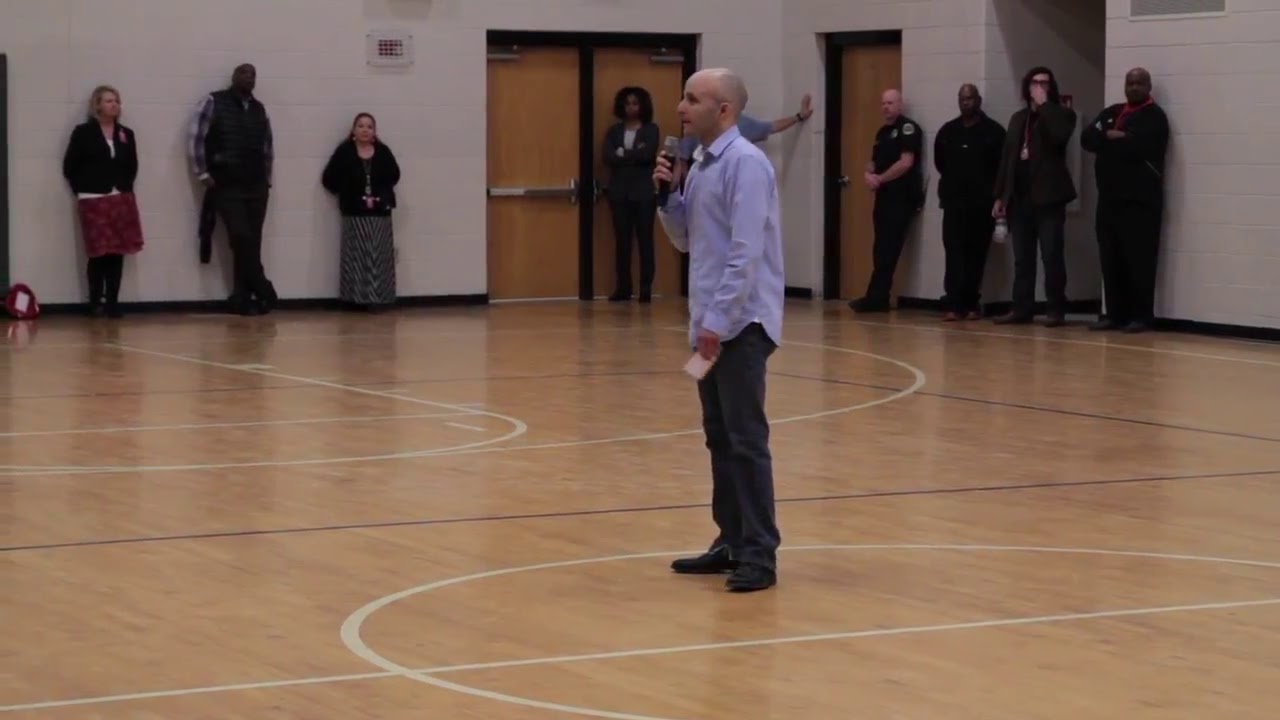The image features a white man in his early 40s, bald, and wearing a blue button-down collared shirt with light black pants and black shoes, standing in the middle of a high school gymnasium. He is making a speech using a microphone. The gymnasium has a wooden floor marked for basketball with white free-throw, three-point lines, and a half-court circle. The background wall is white brick. The man is surrounded by a group of individuals standing along the walls. To his left, there's a woman wearing a red skirt and black top, a tall black man in a dark vest, and an older woman in a long skirt and black top. To the right of this group is a set of gym doors, in front of which stands a black woman. Further to the right, behind the speaker, a man can be seen with only his arm visible against the wall. To the right of this man is another door, beside which stands a white, bald security guard or police officer. Further right, there's a black man dressed in black clothes, a white man with long dark hair and glasses, covering his face, and another bald black man in black clothes. The audience appears attentive, with some crossing their arms or touching their faces.